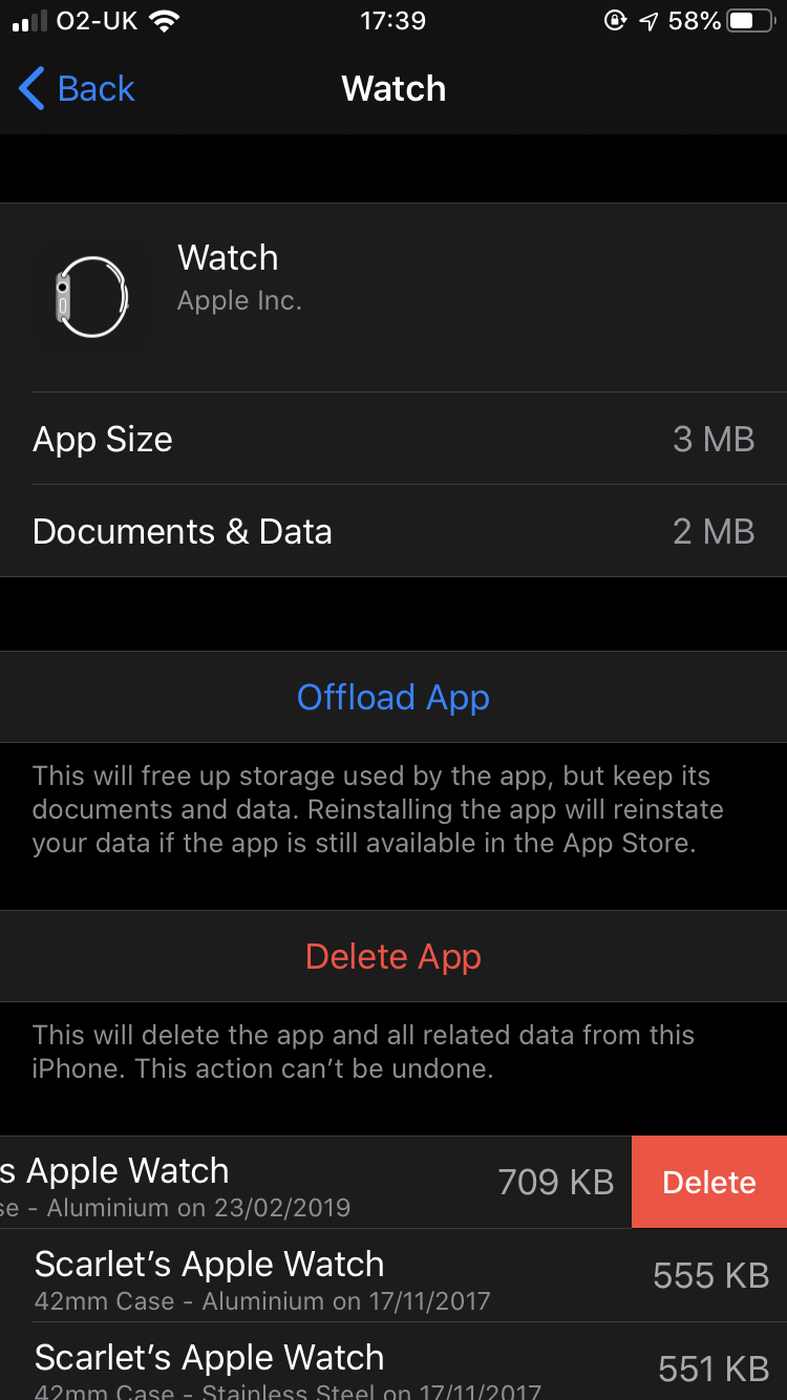This is a detailed screenshot of an Apple Watch settings page displayed in dark mode. At the top of the screen, the word "Watch" is prominently centered in white text. On the upper left, there's a blue "Back" button accompanied by a back arrow icon.

Immediately below, a dark gray section contains the label "Watch Apple Inc." with an image of a watch to its left. This section is followed by two rows, each separated by thin lines, providing specific information about app size and data usage. The first row indicates "App Size: 3 MB," and the second states "Documents & Data: 2 MB."

Further down, there's a blue "Offload App" button that reads, "This will free up storage used by the app but keep its documents and data." Below this, another section features a red "Delete App" button with a warning that states, "This will delete the app and all related data from this iPhone."

At the bottom, under the heading "S Apple Watch," it shows "709 KB" next to a red delete button on the right, providing an option to remove this specific data.